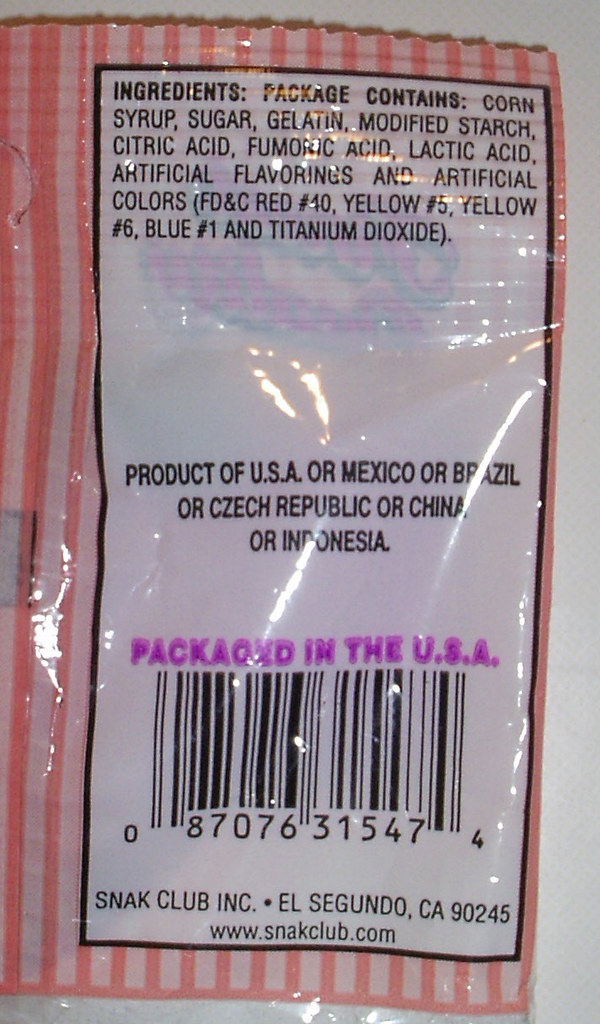The image displays the back side of a plastic packaging, characterized by its highly translucent and almost see-through quality. The packaging is currently empty. The design in the background features vertical pink stripes set against a light pink backdrop. Dominating the center of the packaging is a large white label covering most of it.

At the top of the label, bold text reads "Ingredients" followed by a list of components: corn syrup, sugar, gluten, modified starch, citric acid, lactic acid, artificial flavors, and artificial colors. 

Midway down the label, there's a statement indicating the product's origin: "Product of USA or Mexico or Brazil, or Czech Republic or China or Indonesia." 

Towards the bottom of the label, it clearly states "Packaged in the USA." 

Finally, beneath this text is a standard barcode, complete with various numerical digits beneath it.